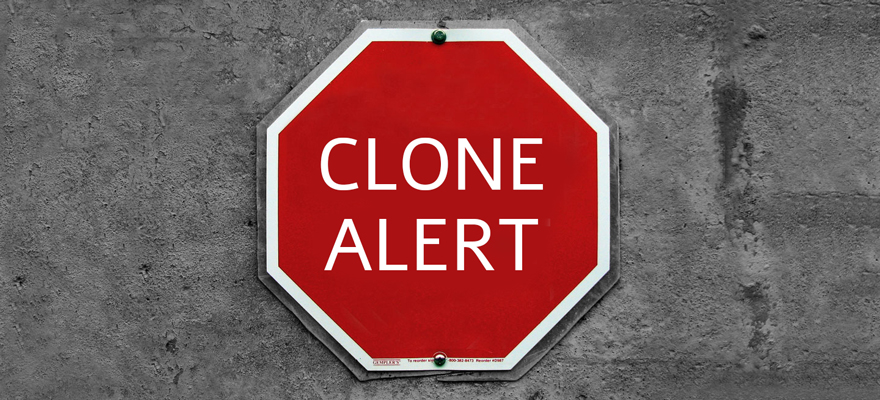The image features an octagonal red sign resembling a traditional stop sign, complete with a white border around its edge. However, instead of the familiar "STOP," the sign displays the words "CLONE ALERT" in bold, white block letters, with "CLONE" on the top line and "ALERT" directly below it. The sign is affixed to a rectangular, dark gray, rough-textured surface, which appears to be concrete or a similarly durable material, using screws or nails at the top and bottom. This concrete-like background is mottled and longer horizontally than it is tall, suggesting it might be part of a wall or a structural element of a building. The exact placement of this sign is unclear, but its unique message prompts curiosity about its intended location and purpose.